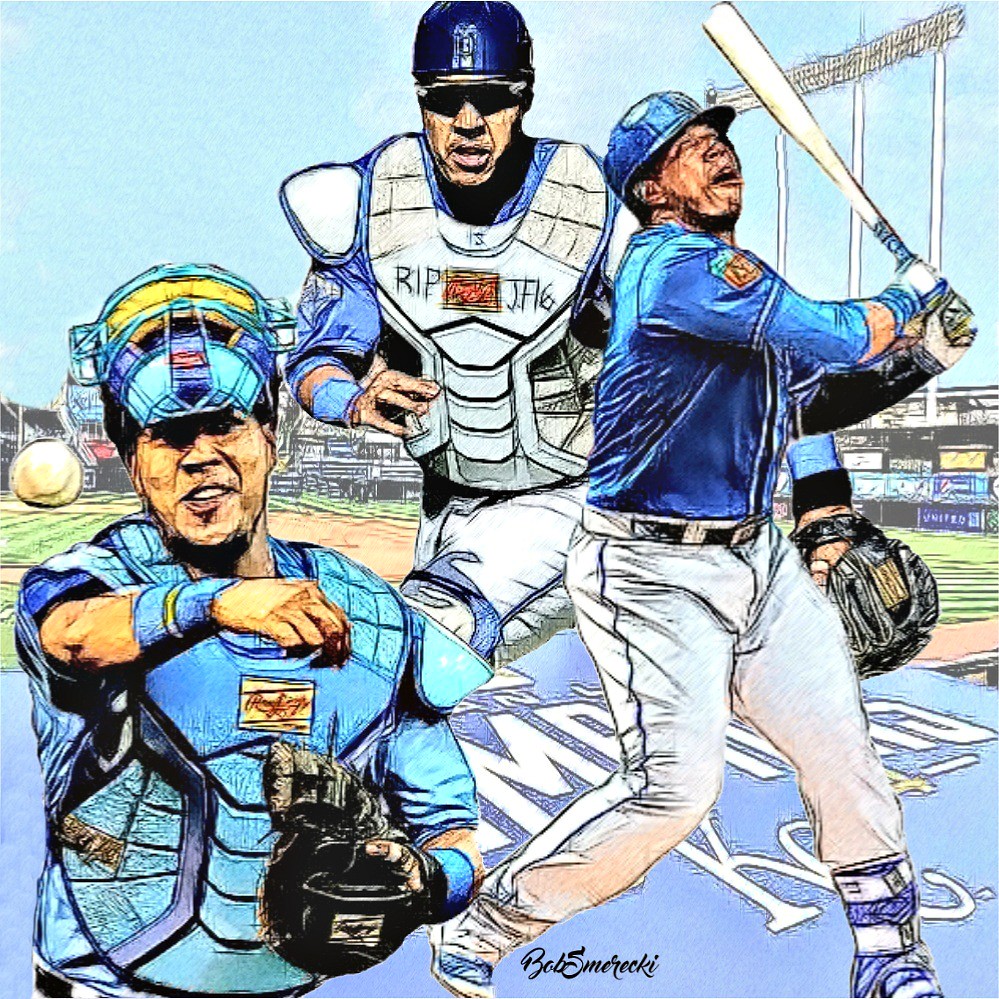This hand-drawn or painted artwork features a central depiction of several baseball players set against the backdrop of a baseball field. The scene is lively and dynamic, with visible details suggesting the presence of floodlights illuminating the sky. The color palette includes a mix of light blue, white, gray, dark blue, yellow, red, and tan, creating a vibrant and engaging visual experience. At the bottom center of the artwork, the name "Bob Smerecki" is prominently displayed, possibly indicating the artist's signature. The intricate details and the artistic style unmistakably point to a handcrafted creation, showcasing the talent and meticulous effort involved in producing this vivid sports-themed illustration.